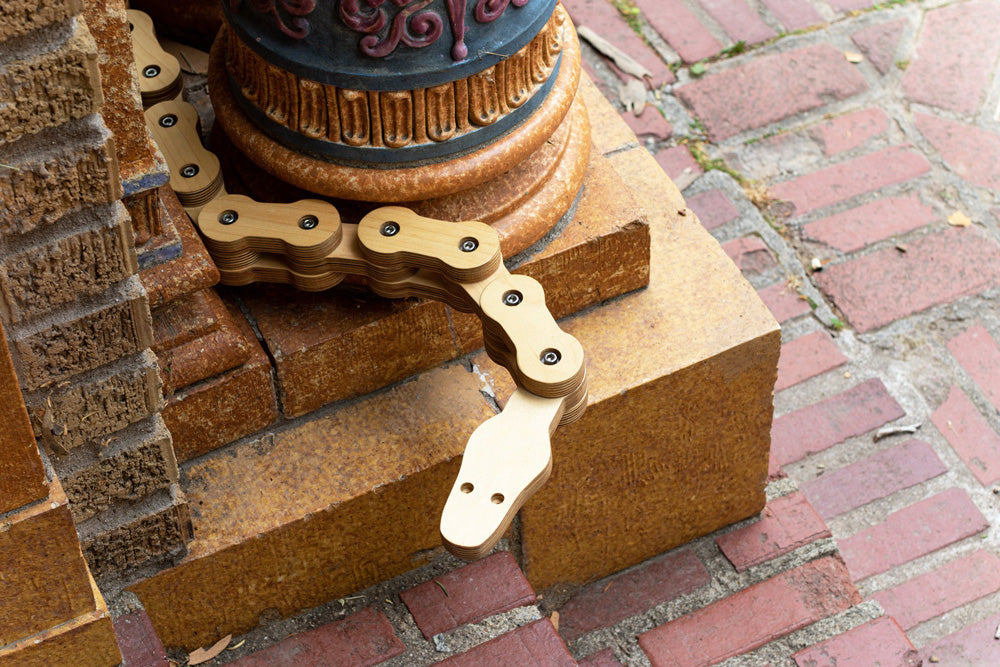The photograph captures a scene featuring a decorative column wrapped by a snake-like wooden toy. The column, circular in shape, displays a multicolored pattern primarily in shades of blue, red, pink, and tan, and is positioned atop a set of tan steps. These steps lead down to a reddish-brown brick sidewalk. The wooden toy, which resembles a snake, is made up of movable wooden links connected by screws at their tops. Each link allows articulation, with the snake's head, complete with two eyes, prominently visible as it curves around the column. The brownish-golden links suggest a wooden material, adding a textured contrast to the vibrant hues of the pillar and the surrounding scene.